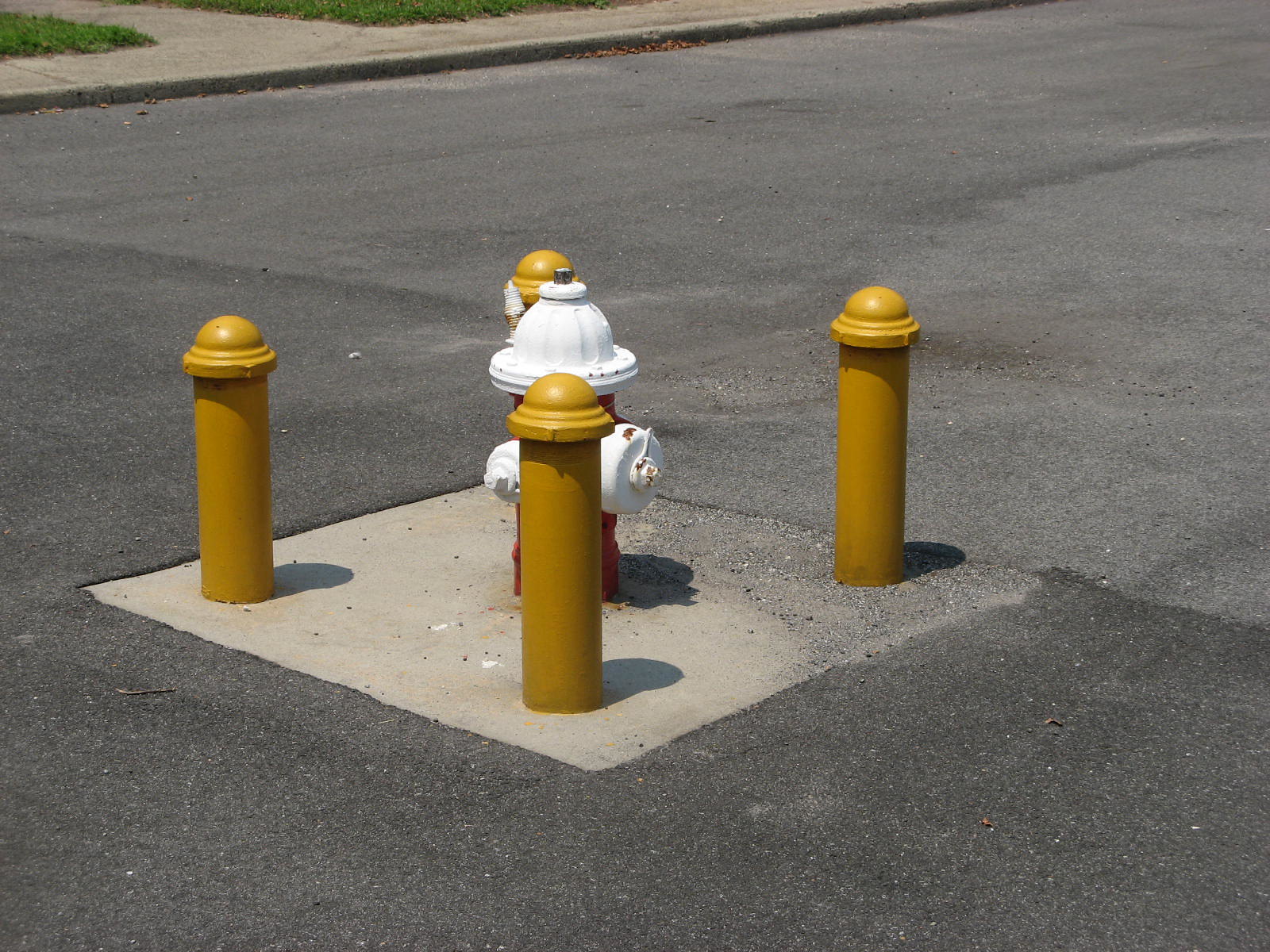An outdoor photograph taken during the day showcases a street scene bordered by vibrant green grass. The image features a well-maintained sidewalk running from the left side towards the upper right, framed by lush grass on both sides. The street, composed of blackish-gray asphalt with areas indicating it has been patched to eliminate potholes, occupies the majority of the image. Toward the bottom left of the scene, there is a red fire hydrant prominently situated on a light gray concrete square in the center of the picture. The hydrant has a white-painted top and white hose connections on both sides, with a small plastic cap at the top. Surrounding the fire hydrant, there are four yellow metal poles, each capped with a rounded top and appearing the same height as the hydrant. Scattered leaves are visible near the curb, adding a touch of natural detail to the urban scenery.